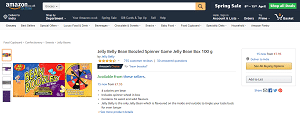The image is a small screenshot from the Amazon website, showcasing a product listing. The distinct black horizontal bar at the top confirms it's from Amazon, with the company's name clearly visible in white font on the upper left corner. Immediately next to it is a large, thin white rectangle serving as the search bar. 

The focal point of the screenshot appears to be a colorful child's game, though the exact details are difficult to discern due to the image's small size. To the right of the game's image, there is a product description written in black text. Below the description, a series of star ratings indicates customer reviews. Further down, a bullet point list outlines key features of the game.

On the left side of the listing, smaller images likely show different angles or components of the game's packaging. On the right side, purchase options are available, with a prominent yellow rectangle indicating the "Buy" button, typical for Amazon. Adjacent to it, a gray button offers additional options such as adding the item to a list or viewing other purchasing choices.